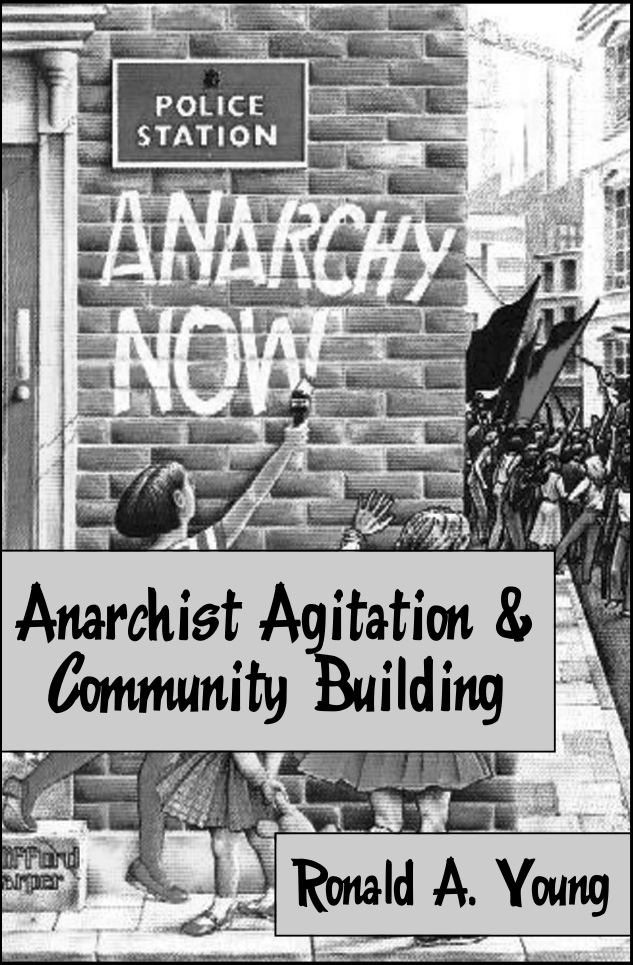The black-and-white illustration, likely a book cover titled "Anarchist Agitation and Community Building" by Ronald A. Young, depicts a chaotic urban scene centered around a brick police station. The brick building prominently displays the sign "Police Station" above a child spray-painting the phrase "Anarchy Now." In front of the building stand three little girls; one holds a paintbrush, another clutches a teddy bear, and the third peeks around the corner, observing a crowd. The street scene to the right features a cluster of people, possibly in the midst of a protest or riot, with indistinct outlines of other buildings in the backdrop. The gray banners with black lettering serve as striking focal points in the composition, highlighting the book's title and author.